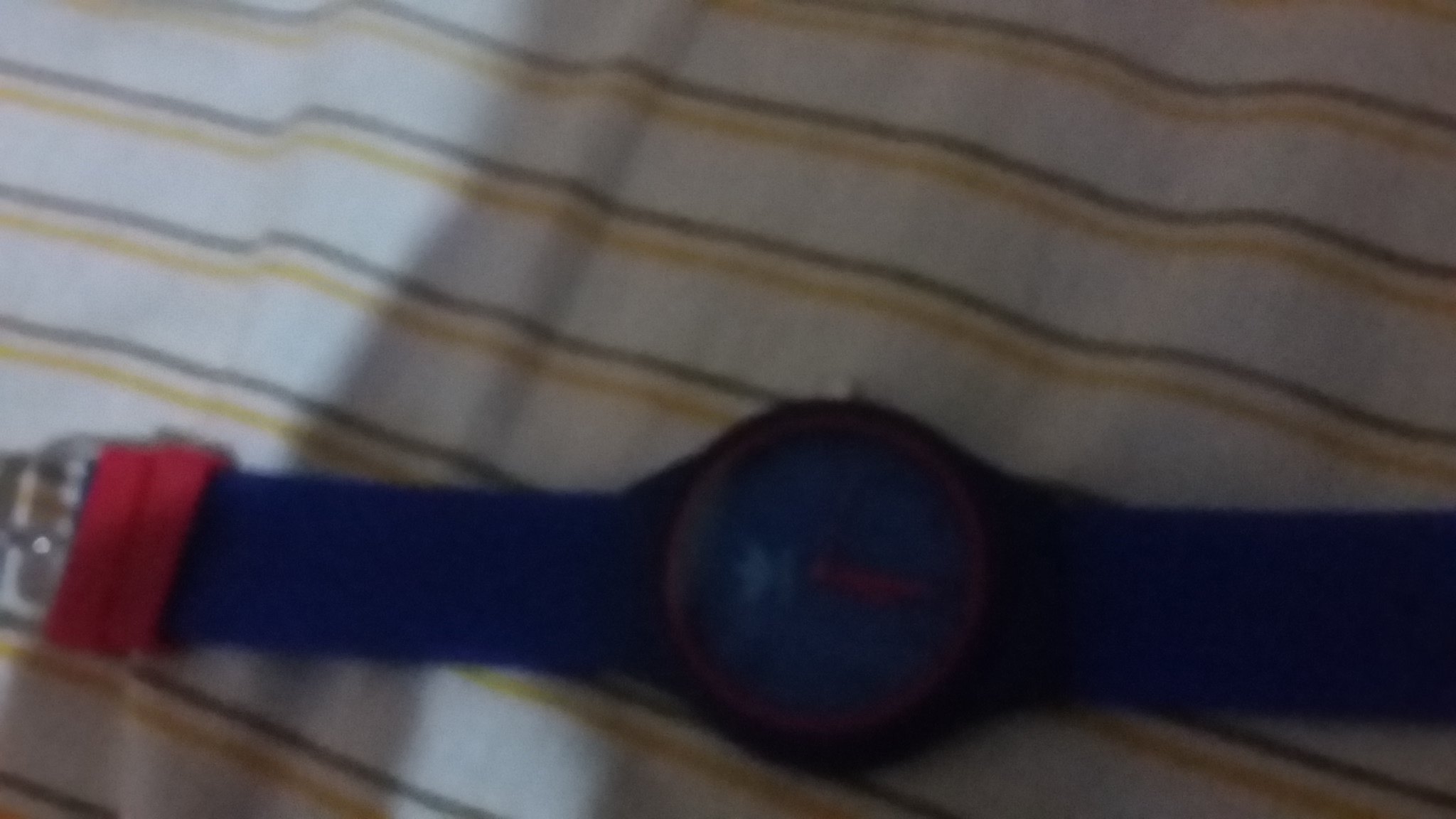This is a blurry, vintage-looking photograph that appears to be an older image. The focus of the picture is a child's watch, lying horizontally on a white, vintage-striped bedsheet. The sheet features distinctly thick white stripes complemented by thinner yellow and brown stripes. The watch itself has a dark blue band with a matching blue face. Though somewhat indistinct, the face seems to bear an Adidas logo. The watch hands are red, adding a vivid touch to the design, while a black circle frames the face. Additionally, the buckle, where the band is secured, stands out in a bright red hue.